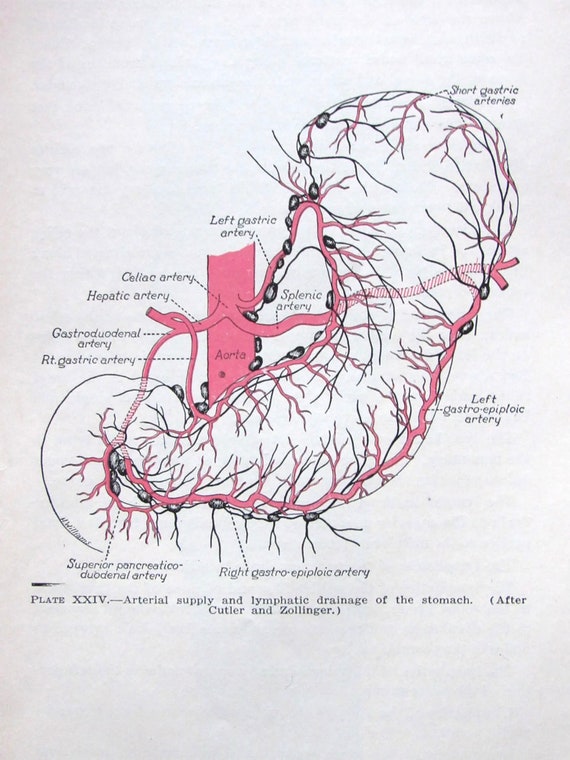The image depicts a detailed medical diagram of a stomach, resembling an illustration from a textbook. The stomach, centrally located and shaped akin to a kidney bean, is intricately drawn and filled with numerous vein-like structures, some black and others red. These structures are primarily arteries, annotated with black text outlining various parts of the stomach’s arterial and lymphatic system.

Key annotations at the top include "Short Gastric Arteries," and notable labels within the diagram identify the "Left Gastric Artery," "Splenic Artery," "Left Gastroepiploic Artery," "Superior Pancreaticoduodenal Artery," and "Right Gastroepiploic Artery," among others. The pink lines, extending to and from these arteries, add a distinct layer of detail and mimic real biological structures connecting to the aorta and other major vessels.

The bottom of the diagram features the caption "Arterial Supply and Lymphatic Drainage of the Stomach," followed by "after Cutler and Zollinger" in black text, suggesting the image's reference source. The overall background is an off-white color, lending a vintage appearance to the entire illustration. The meticulous rendering of the arteries, combined with the precise labeling, reflects the diagram’s intent to provide a comprehensive view of the stomach's blood supply.